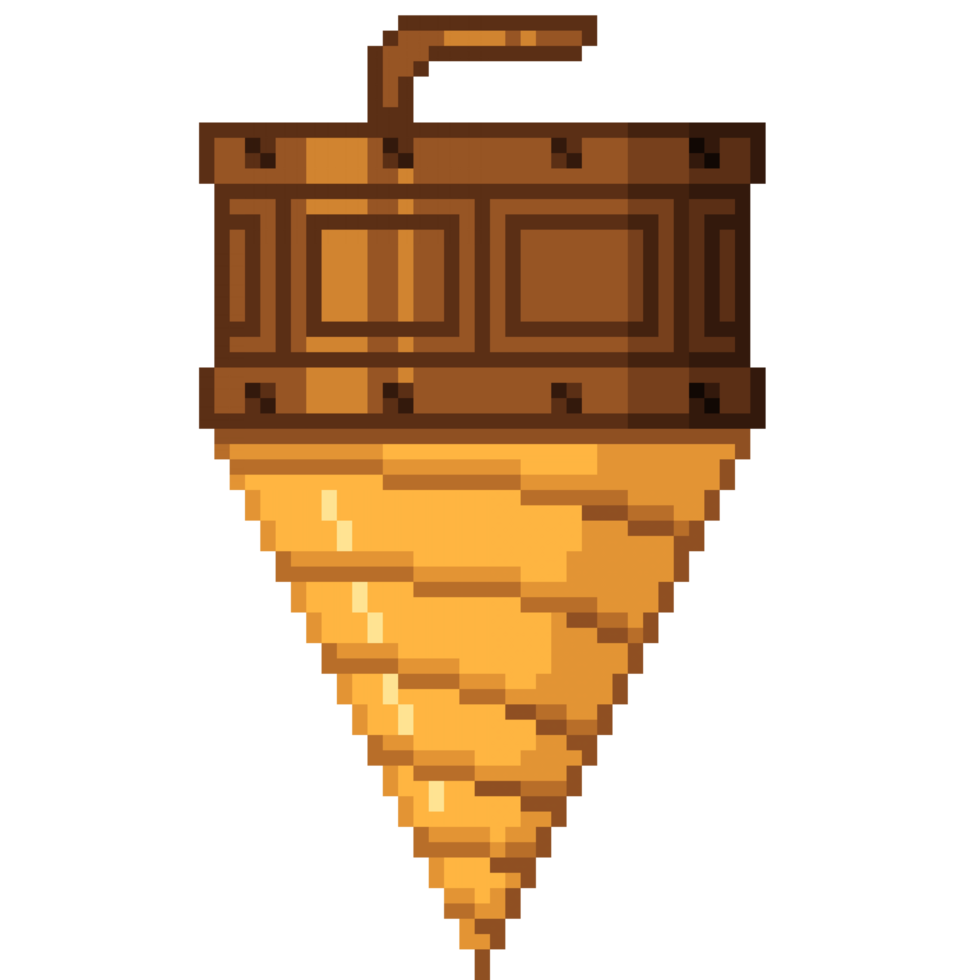The image depicts an artistic rendition of a funnel-like structure set against a white background. The object resembles a pencil point but is actually a drill bit-like form. The bottom part of the object is funnel-shaped, predominantly yellow and golden with lighter yellow specks, while the upper part is primarily brown, dark brown, and contains black outlines. A lever or clasp is situated at the top, adorned with multiple dots and squares, and resembles a vent. There is also a small basket-like feature attached. The entire structure looks like it could be tunneling into the ground, with around six distinct lines indicating this action. There is no textual information present in the image.